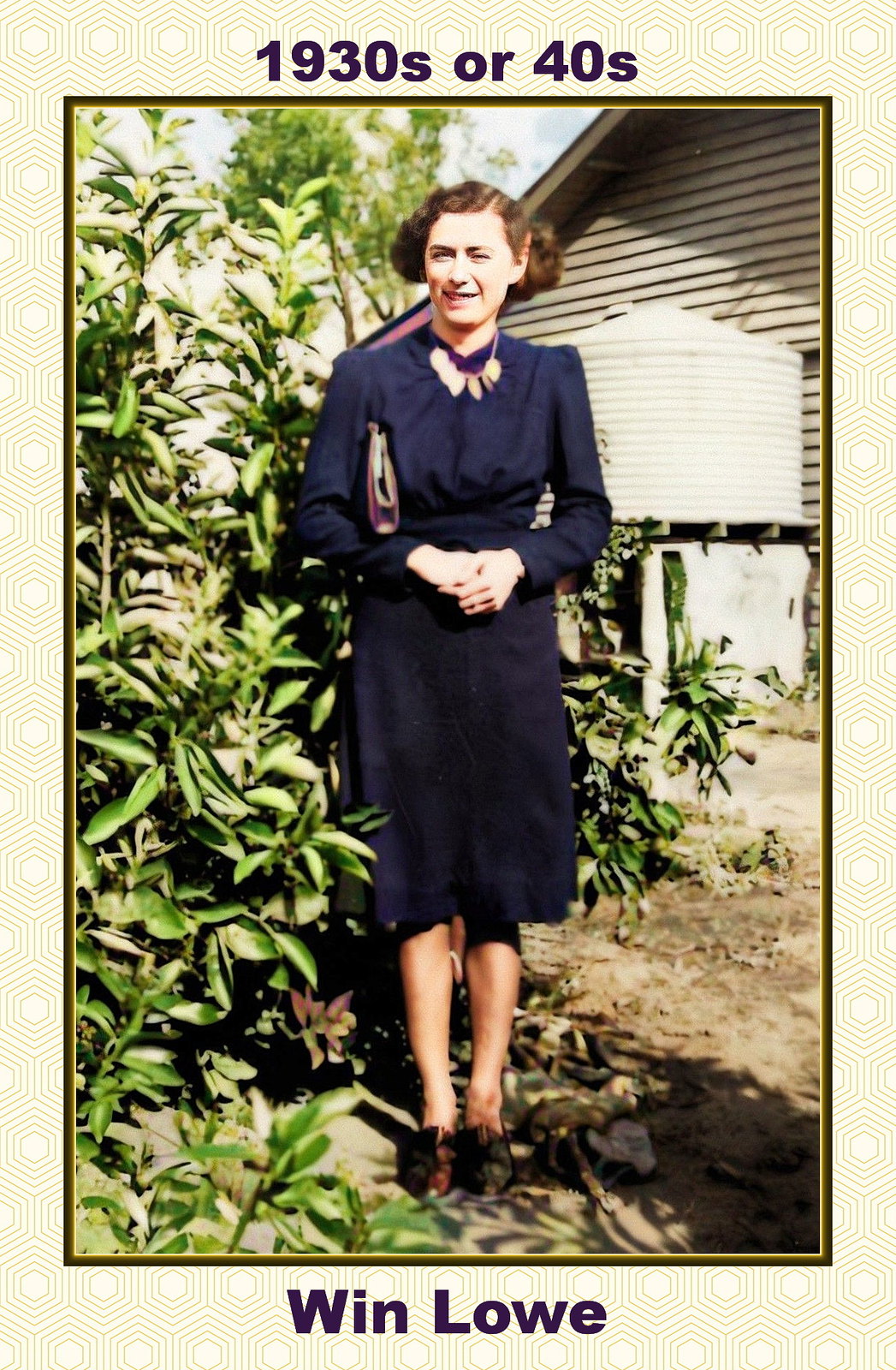An old, colorized photograph from the 1930s or 40s, as indicated by text in a black font at the top, captures a white woman posing outdoors. She stands confidently in a garden or farm-like setting, in front of a large rhododendron bush to her left and a house and water cistern to her right. The photograph is framed by a thick border with lines, circles, and geometric designs, transitioning to a thin black border, and finally a slimmer gold border. The woman, with short, slightly curly brown hair, wears a long-sleeve dark blue shirt and a black knee-length skirt. She accessorizes with a necklace, brown shoes, and holds a pocketbook under her left arm. Her hands are clasped, and she offers a subtle, half-smile to the camera. Below the photograph, in the same black font, is the name Win Low.